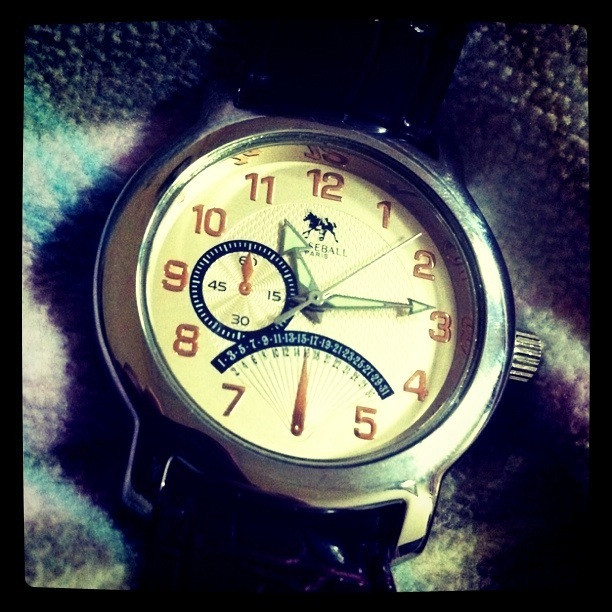This is a detailed close-up photograph of a wristwatch with a traditional dial and hands, resting on a soft, multi-colored material that might be a blanket, tablecloth, or rug, featuring shades of white, light blue, and dark blue. The watch has a stainless steel silver bezel and winder, and a black strap that appears in shadow. The watch face is cream-colored or very light yellow, and it prominently displays the numbers 12, 1, 2, 3, 4, 5, 7, 8, 9, 10, and 11 in red. The number 6 is replaced by a red pointer, which is part of an arc that includes the numbers 1 to 31, likely indicating the date. The face also features a smaller blue-ringed circle near the number 9, marking 60, 15, 30, and 45 seconds. The time on the watch is approximately 11:14, with luminous green hour and minute hands that also note seconds. There is an image of a galloping horse, and the partially obscured brand name appears to read "S-E-B-A-L-L Paris."